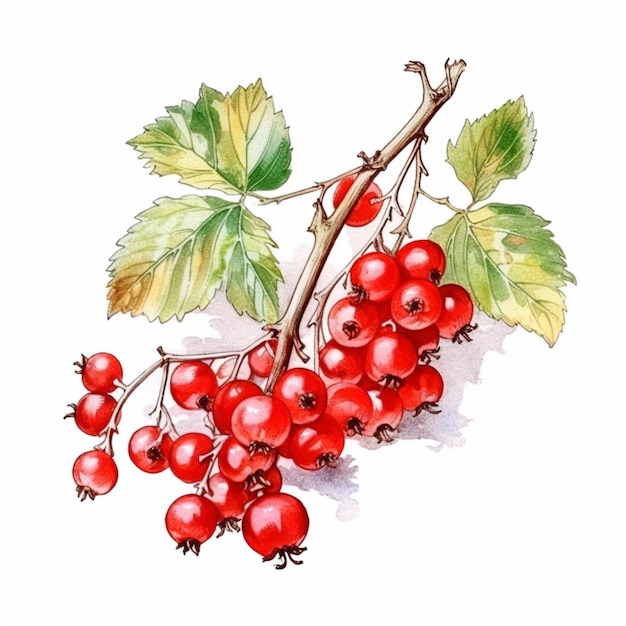This is a detailed illustration depicting a cluster of bright red berries that resemble cherries but also share characteristics with persimmons and cranberries. The berries, which are vividly red with white highlights, hang in tight bunches from a brown woody vine that branches out in multiple directions. Some clusters hang together, while there is one solitary berry near the top. The green and yellow leaves, with varying shades and patches of color, including a bit of brown on one of them, add a natural touch to the image. The overall rendering is stylized and artistic, reminiscent of vibrant fruit illustrations you might find on the side of a fruit box. The background is absent, emphasizing the meticulous detail and freshness of the fruit and foliage.